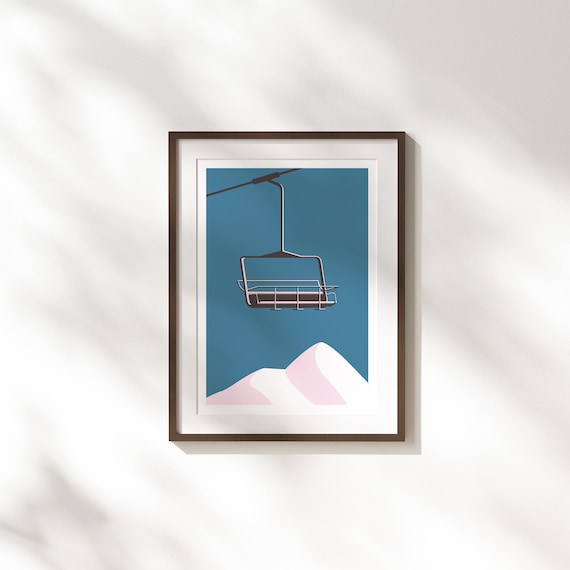The artwork depicted is a stylized and detailed painting of a ski lift, framed elegantly and displayed against a wall that appears cloud-like with hues of white and gray. Encased in a black frame with an off-white mat border and a thin inner white frame, the painting captures a single ski lift suspended from a cable that is depicted in black. The ski lift itself, shown without occupants, is composed of black and white shades, featuring a seat with a safety bar across it. Below the lift, the painting illustrates a scenic mountain with white peaks and hints of pink and gray, creating a serene contrast against a vivid blue background. The overall effect is of a solitary ski chair hovering above an artfully rendered winter landscape.